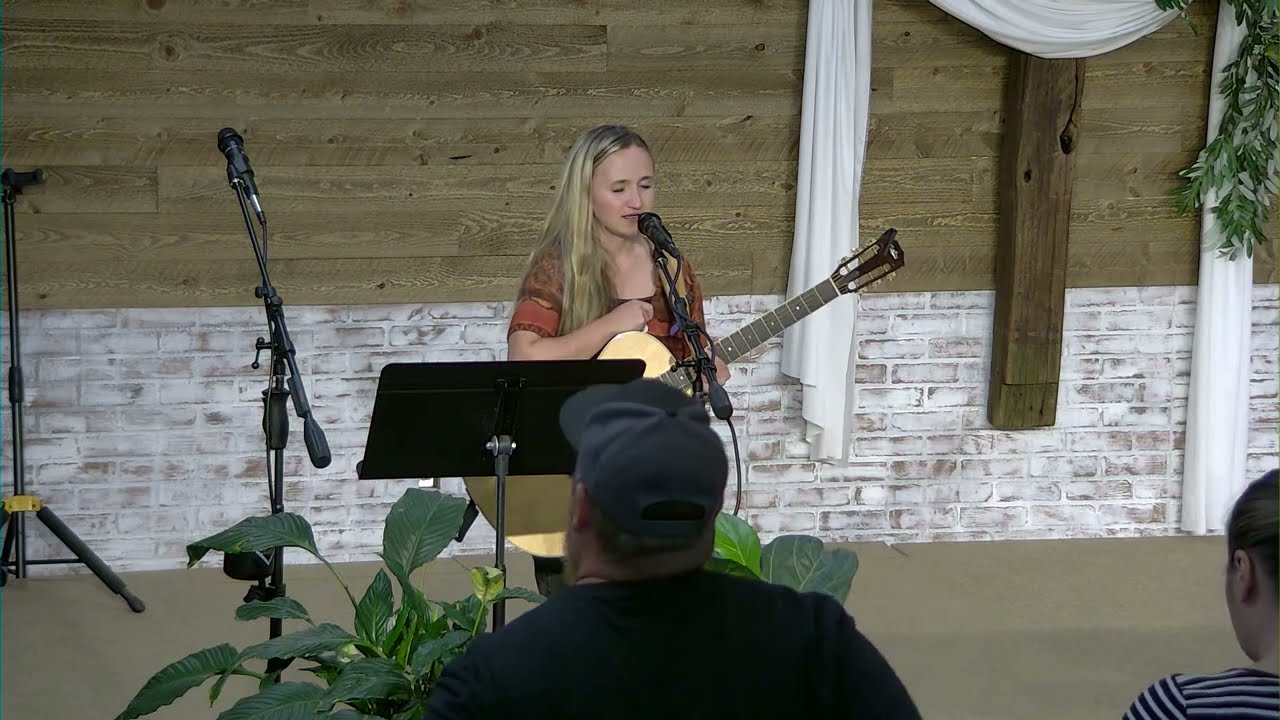In a detailed and well-composed landscape photograph, a young woman with light skin and long blonde hair, cascading below her shoulders, stands at the center behind a black podium. She is speaking or possibly singing into a microphone, her eyes closed in concentration. Dressed in a light red blouse with sleeves ending just above the elbow, one of her arms is raised, hand near her chest. A yellow acoustic guitar with a black neck rests in her hands, suggesting a musical performance. 

The stage she occupies is set against a striking backdrop: the upper half is wooden, the lower half features weather-beaten, white-painted brick, with a strip of wood down the center. To her right, a curtain is drawn open. There is also a partially visible wooden cross draped with white cloth, indicating a setting that resembles a church. An additional, unoccupied microphone stands to her left along with a black music stand.

In the foreground, a man with his back turned—wearing a black cap and jacket or shirt—faces the performer. Nearby, another person in a black-and-white striped shirt sits with their head bowed. A lush green plant with large leaves adds a touch of nature to the otherwise serene and intimate stage setting. The ground is a light, clean gray, and some vegetation hangs from the upper right corner, completing the scene with a touch of natural serenity.